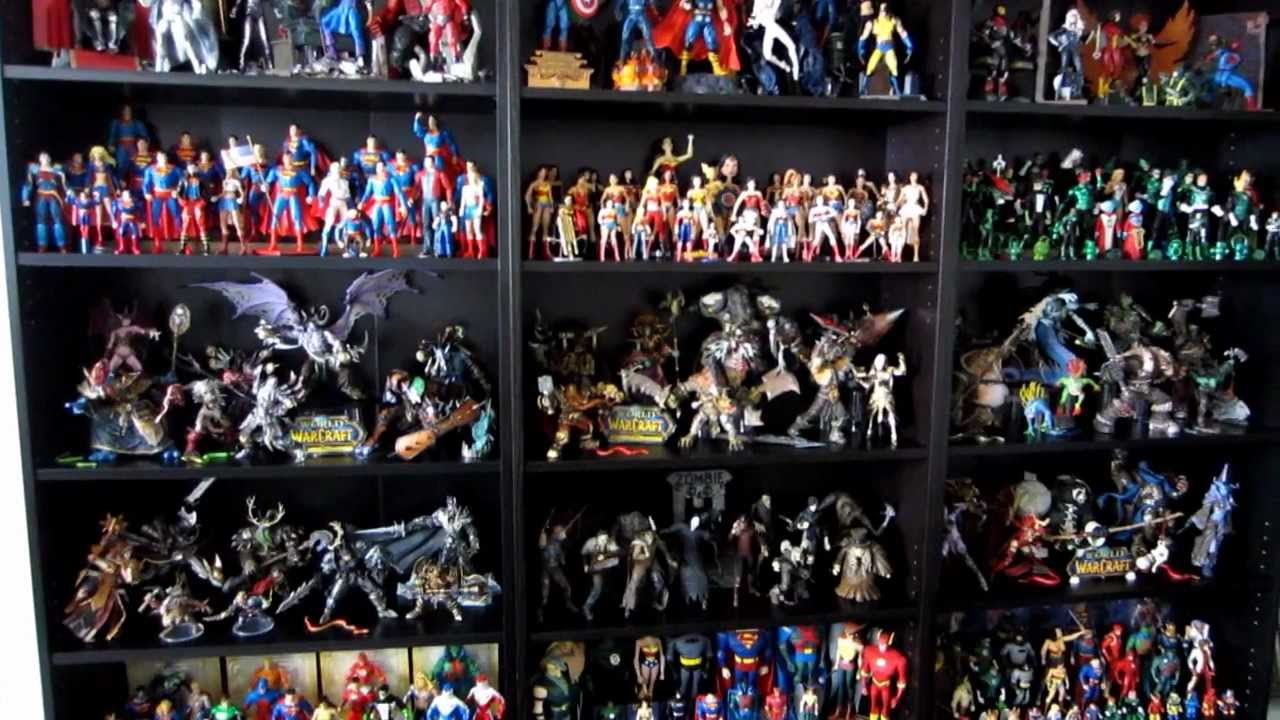The image showcases a black shelving unit, possibly composed of three vertical cabinets placed side-by-side, each with multiple shelves. The shelves are densely packed with a wide array of small, plastic action figures that represent various iconic characters, primarily from science fiction and fantasy genres. On one entire shelf, there is a dedicated collection of Superman figures, easily identifiable by their classic blue suits, red capes, and red underwear over blue pants. Another shelf displays an array of superheroes, including recognizable figures like Batman, Spider-Man, and Batwoman. Additional shelves feature diverse assortments of characters, from Power Rangers to dragons, and even some more intimidating figures, such as a character with a big bat. There are also rows with Wonder Woman and other fantastical figures. The organization of the shelving suggests a thematic grouping, though some figures appear scattered, indicating that meticulous categorization might not have been the priority. The top shelf is partially cut off in the image, adding to the expansive view of this impressive collection.